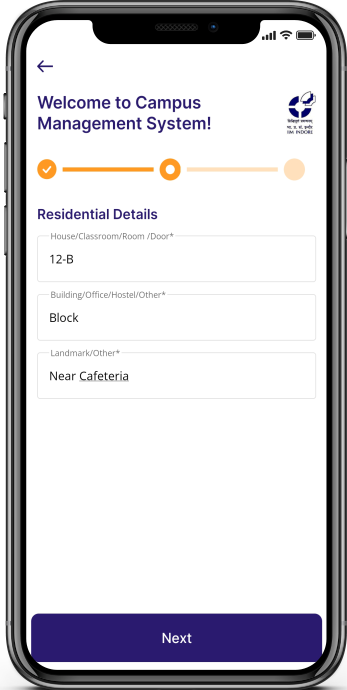In the image, a smartphone screen displays the interface of the Campus Management System. At the top of the screen, a header reads "Welcome to Campus Management System." Below the header is a progression bar illustrating the user's progress, highlighted with an orange check mark indicating completion of the current step.

Under the progression bar, the label "Residential Details" is prominently shown. Beneath this label are three text input boxes, each with designated titles and filled entries. The first input box is titled "House/Classroom/Door," containing the text "12-B." The second input box, labeled "Building/Office/Hostel/Other," has the entry "Block." The third and final input box, titled "Landmark/Other," contains the text "Near Cafeteria."

At the bottom of the screen, there is a prominent purple navigation button labeled "Next," which likely advances the user to the subsequent step in the system's setup. In the top-right corner of the screen, standard icons indicate the battery level and navigation status, providing essential information about the cell phone's connectivity and power.